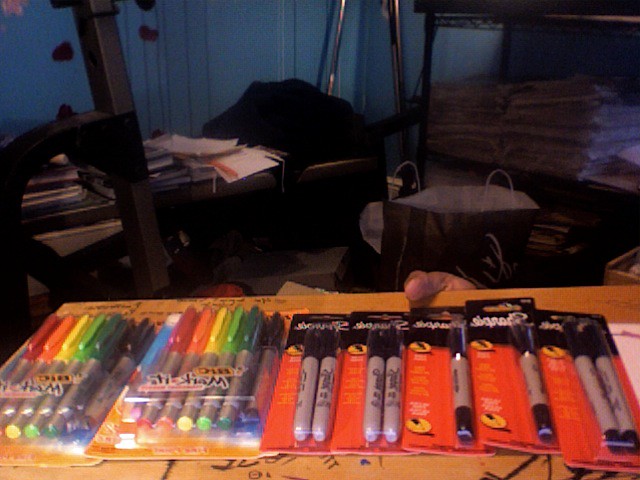This color photograph captures a cluttered indoor setting, showcasing a scene dominated by various packages of markers spread across a surface. The image quality is poor, adding to its chaotic impression. In the foreground, we see a surface that might be a cardboard box or a brown wood table. Resting on it are a total of seven marker packages. 

On the left side, there are two packages of Bic markers in a spectrum of colors including red, orange, yellow, green, blue, and turquoise. To the right, there are five packages of Sharpie markers, each featuring two black permanent markers with distinct gray bodies and black lids, set against an orange cardboard backing.

Towards the bottom edge of the photo, a thumb is visible, seemingly holding up the piece of cardboard or the table, anchoring the scene in a casual snapshot manner. The background reveals more disarray with piles of papers on a table and items stacked on a steel shelf, all set against a light blue wall that enhances the sense of a neglected, busy environment.